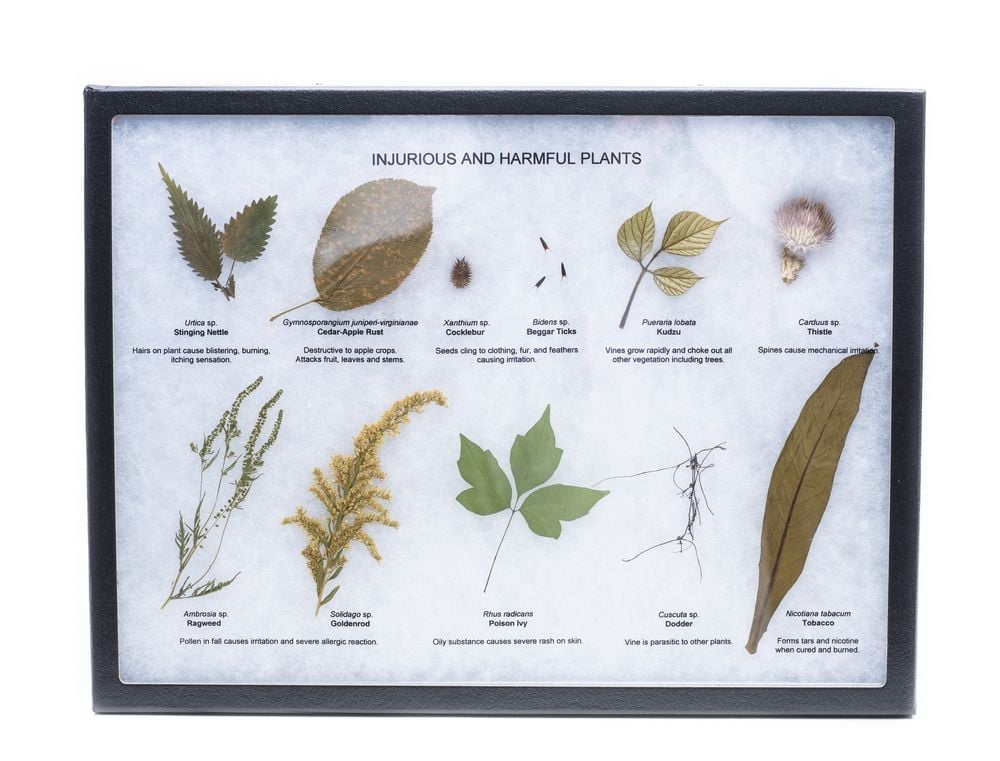The image features a vividly detailed scientific illustration titled "Injurious and Harmful Plants," set against a clean, white background and framed in black. Within this frame, a variety of plant species are displayed, each labeled with their scientific name and the harmful effects they cause.

Prominently featured plants include:

1. **Urtica sp. (Stinging Nettle)**: Recognizable by its zigzag-shaped leaves, this plant’s hairs cause blistering, burning, and itching sensations.
2. **Gymnosporangium juniperi-virginianae (Cedar-Apple Rust)**: A plant pathogen destructive to apple crops, affecting fruit, leaves, and stems.
3. **Xanthium sp. (Cocklebur)**: Notable for its bur-like seeds that cling to clothing, fur, and feathers, causing irritation.
4. **Bidens sp. (Beggarticks)**: Similar to Cocklebur, its seeds adhere to various surfaces, causing irritation.
5. **Pueraria montana var. lobata (Kudzu)**: Illustrated choking out other vegetation, including trees, due to its rapidly growing vines.
6. **Cirsium sp. (Thistle)**: Known for its spines that cause mechanical irritation.
7. **Ambrosia sp. (Ragweed) and Solidago sp. (Goldenrod)**: Both plants produce pollen in the fall that can cause severe allergic reactions.
8. **Toxicodendron radicans (Poison Ivy)**: Its stem contains an oily substance that results in severe rashes.
9. **Cuscuta sp. (Dodder)**: Depicted as a parasitic vine detrimental to other plants.
10. **Nicotiana tabacum (Tobacco)**: Displays a large brown leaf; when cured and burned, it forms tar and nicotine.

This organized, text-rich image—with clear captions denoting each plant's name and harmful effects—resembles a page from an academic textbook or a scientific presentation.